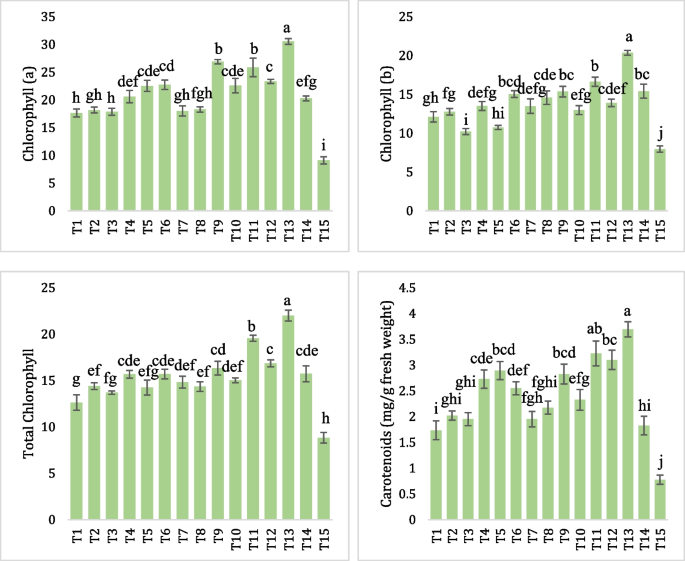The image displays a four-panel presentation of bar graphs arranged in a grid with two charts on the top row and two on the bottom row. Each bar in the graphs is a pale green color. None of the graphs have titles. All four bar graphs feature an x-axis labeled from T1 to T15. 

The bar graph in the top left corner is labeled "Chlorophyll A" on the y-axis, which ranges from 0 to 35 in increments of 5. Adjacent to it on the top right is the graph for "Chlorophyll B," with a y-axis ranging from 0 to 25, again in increments of 5. Moving to the bottom left, the graph is labeled "Total Chlorophyll," with its y-axis spanning from 0 to 25 in 5-point intervals. Lastly, the bottom right graph denotes "Carotenoids (Mg/G fresh weight)," with a y-axis extending from 0 to 4.5 in 0.5-point increments.

These bar graphs likely represent varying levels of different chlorophyll types and carotenoids in a studied substance, formatted for a scientific audience familiar with the subject matter. While the exact measurement units for chlorophyll concentrations aren't specified, the consistent formatting and labeling suggest comparative analysis across different types.